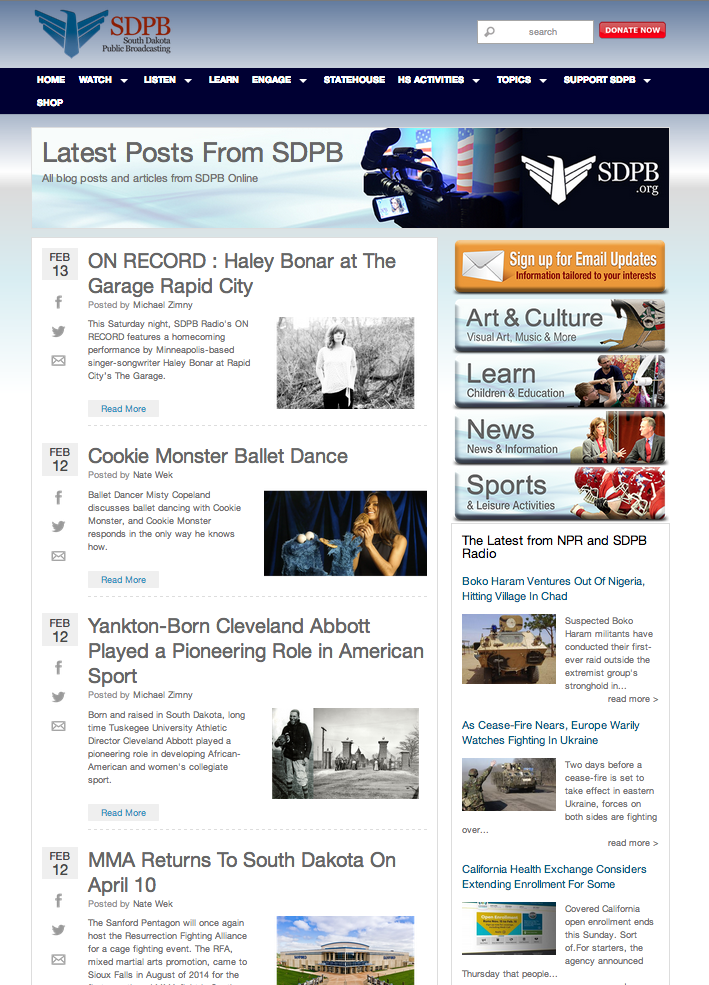The image is a screenshot taken from the website SBPB.org, a public broadcasting site. In the top left-hand corner, the website's logo is visible, featuring an illustration of a bird with open wings. The top right-hand corner includes a small search bar adjacent to a prominent red button labeled "Donate Now" in white text.

The webpage showcases a variety of articles, predominantly related to musical events and concerts. Notable articles include "Cookie Monster Ballet Dance" and "On Record: Hayley Bonner at The Garage, Rapid City." An email sign-up option is also available in the upper right section for users to receive updates.

Each article is accompanied by an image that visually represents its content, and publication dates are displayed beside the articles. The website interface is designed to offer easy access to various articles and blog posts, enhancing the user experience on SBPB.org.